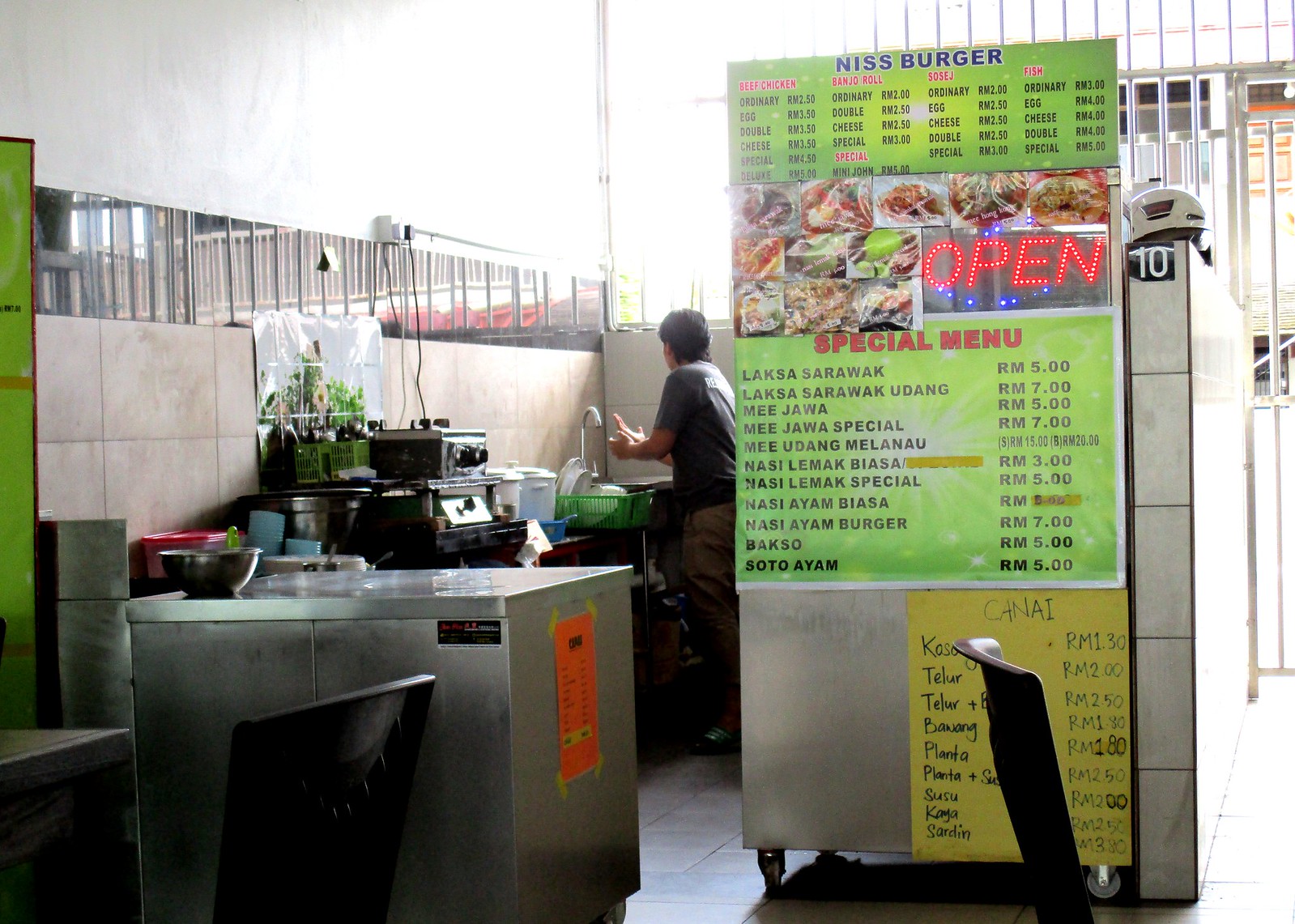This detailed photograph captures the kitchen area of a restaurant, possibly named Nis Burger, which features both indoor and open-air elements. On the left side of the image, a man is standing by a kitchen sink, washing his hands or dishes, next to a stainless steel tabletop that likely doubles as a refrigerated storage cabinet. The cream-colored tiled wall behind him has a long window that lets in natural light, illuminating the various kitchen instruments and utensils neatly organized on a nearby shelf. 

On the right side, a brightly colored menu with a lot of green stands out, listing multiple dishes and their prices in an Asian language. Notable items include "Laksa Sarawak" priced at RM5, "Laksa Sarawak Udang" at RM7, "Nijawa" for RM5, and the "Nijawa Special" for RM7. Below this main menu, there's a yellow, handwritten menu attached to a stainless steel appliance, possibly a refrigerator. In the foreground, several chairs suggest the presence of a dining area nearby. The background of the image features a brighter, possibly outdoor section, with gates indicating an open-air environment that's bathed in sunlight. The overall ambiance strikes a balance between functionality and a clean, inviting atmosphere.